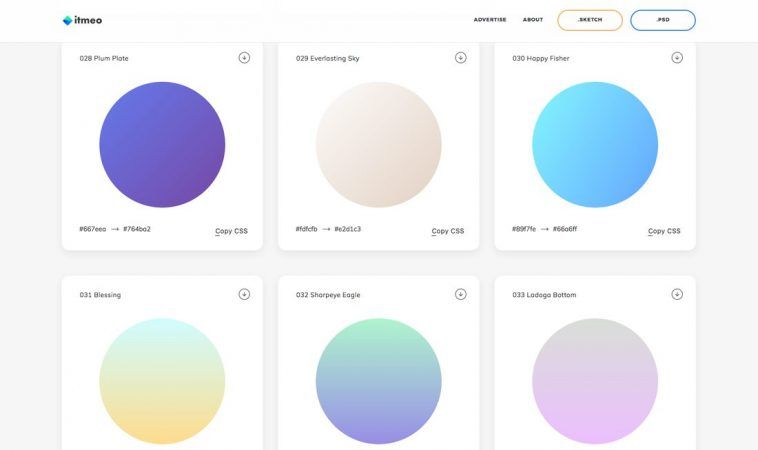**Descriptive Caption:**

The image is a screen capture of a color selection menu interface. At the top left corner, there is a small logo, followed by the text "ITMEO." To the right of the text are menu items labeled "Advertise" and "About." The option "Sketch" is highlighted within an oval button with a light brown outline, while the ".psd" button next to it is outlined in blue, both buttons having a white background.

Below this menu, there are six boxes arranged in two rows, each with a white background. The first box on the top left is labeled "028 Plum Plate," though the text is somewhat fuzzy. Each box has a small down arrow on the right side. At the bottom left of this section, there are two pairs of color codes: "#667EEO" and "#764B02." Next to "Plum Plate," the other color names in the top row are "Everlasting Sky" and "Happy Fisher." The bottom row contains additional color options, though they are not specified in the description.